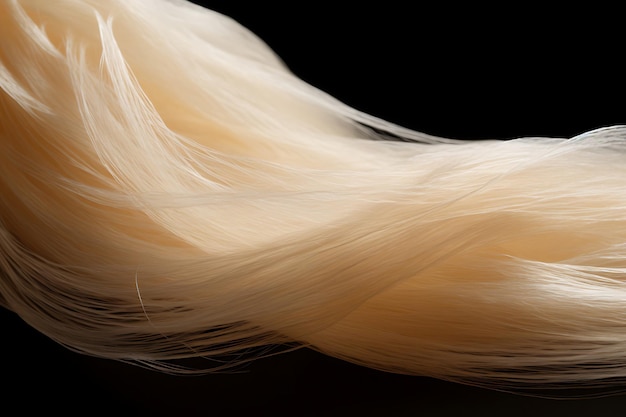This highly detailed, color photograph captures an extreme close-up of a delicate, cream-colored textile. The material, likely a sheer, flowing fabric or possibly spider silk, extends diagonally from the bottom right to the top left of the image in a soft, wave-like curve. The fabric's gossamer-thin fibers are almost transparent, contributing to its lace-like appearance despite lacking traditional lace stitching. The strands exhibit a light blonde, almost platinum hue, with reflective highlights that add a touch of shine, enhancing the material's decorative quality. The background is a deep, solid black, providing stark contrast and emphasizing the fabric's intricate, translucent details. The image is a striking example of photographic realism, focusing intently on the fine textures and subtle variations in color and light of the fabric.